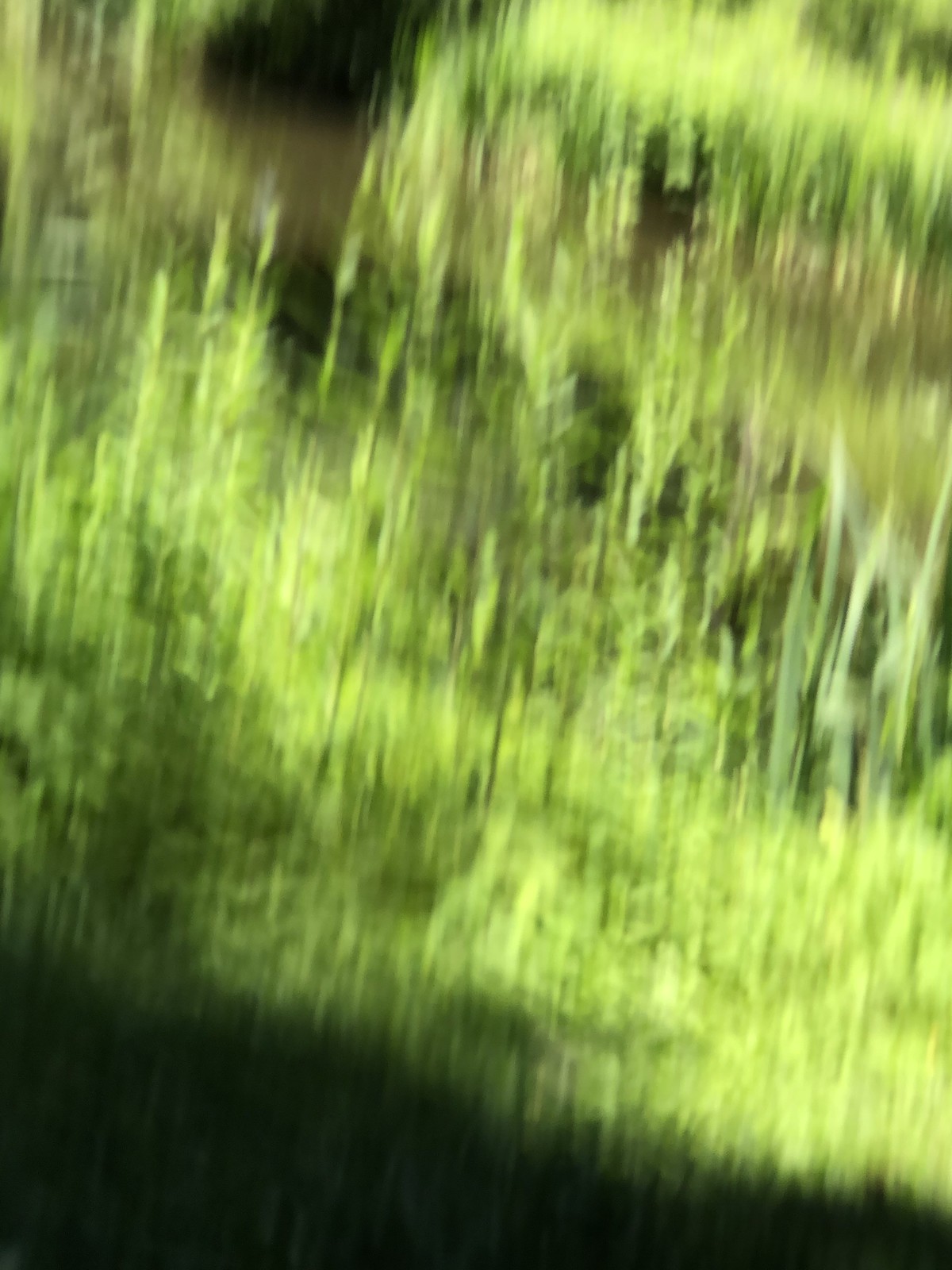This image is extremely blurry, making it difficult to discern specific details clearly, but it captures a swampy area rich in green vegetation. Tall grasses and slender-stemmed plants dominate the scene, with some appearing to be creeping plants hanging from above. The image also reveals a tree in the top right corner with lush green leaves. The center and lower sections of the image are filled with dense green plants and vegetation, some of which resemble weed-like bushes. There is a notable dark black shadow spanning from the bottom left to the bottom right corner, obscuring some of the green vegetation. In the top center of the image, there appears to be a body of water—possibly a muddy river, lake, or stream. Across this water, more green vegetation and trees can be seen, adding to the lush, natural ambiance of the scene. The overall color palette includes various shades of green, some tannish brown from the muddy water, and areas of black from the shadows.